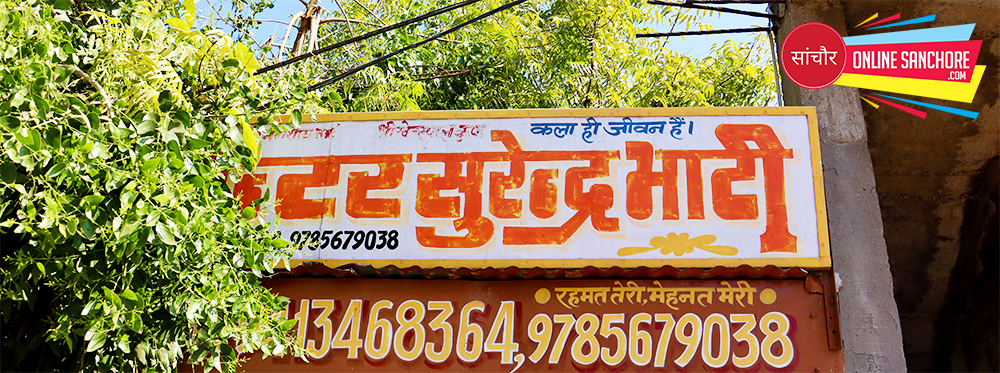The image depicts two signs mounted on a wooden telephone pole, positioned outdoors amidst vibrant greenery and telephone wires. The upper sign features white text on an orange background, written in Hindi, and includes the numbers 9785679038 and 13468364 in blue at the bottom. Below this sign is another in brown with slightly dirty white or yellow numbers. Both signs extend outward from the pole to the left. A distinctive logo appears in the upper right corner of the image: a red circle with Hindi text, accompanied by a red ribbon banner declaring "onlinesandshore.com" in white font, and flanked by ribbons of various colors including yellow, turquoise, and blue. The backdrop reveals lush green tree leaves and a clear sky, reinforcing the image's setting in India.